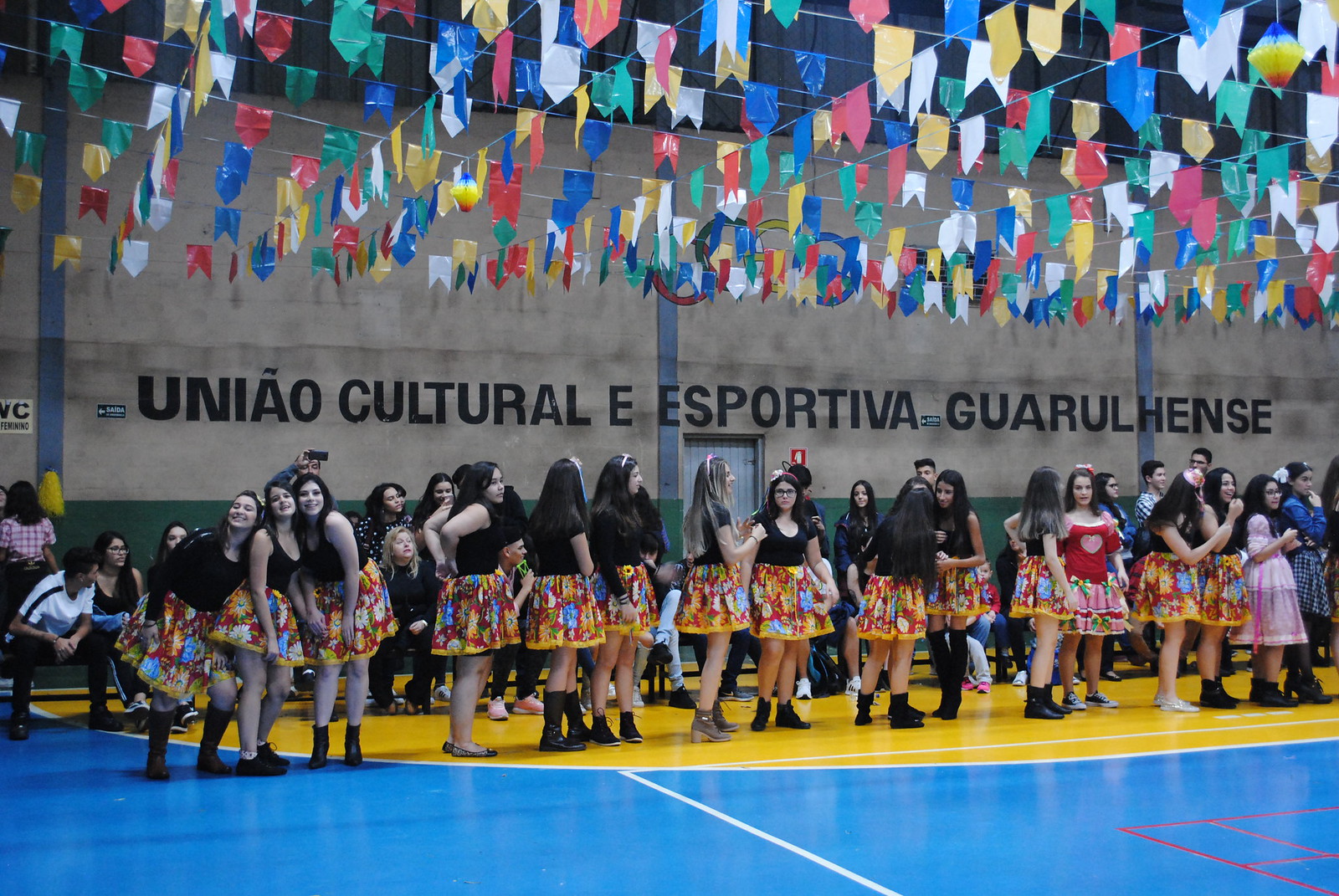The vibrant photograph captures a lively cultural meet-up held in a sports hall decorated with an array of colourful pendant flags strung in a criss-cross grid from the ceiling. Predominantly young women form a line across the blue and yellow marked floor, wearing brightly coloured, floral-patterned skirts reaching above their knees and black sleeveless tops, with a few exceptions donning different coloured tops or dresses. The floor's shiny surface gleams under the overhead lights, revealing white, red, and yellow grid markings typical of a sports hall. Behind the group, some individuals are seated on benches, adding to the community feel of the event. The name “Unio Cultural Esportiva Gurelenza,” painted on the grey back wall, suggests a cultural background, possibly Portuguese, reinforcing the event’s theme. The women in the foreground appear to be enjoying themselves, chatting, and posing for photos, adding a sense of camaraderie and celebration to the scene.